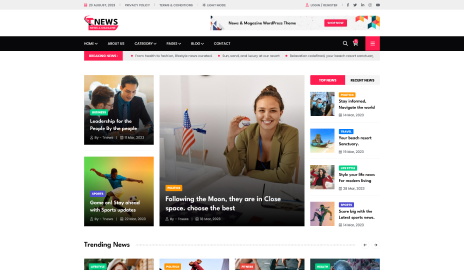The image features a gray banner at the top, though the text is too blurry to read. On the right side of this banner, there are icons for Facebook, Twitter, and LinkedIn, as well as other icons that are indiscernible. Below the gray banner, the word "news" appears in black text with a pink "T". Beneath this, there's a pink banner, but its text is unreadable. Next to this pink banner on the right, another gray banner contains some black text, although it's also too blurry to decipher. 

Further down is a black banner with the word "home" clearly visible, followed by other words that are blurry, except for "category." Towards the far right of this section, there's a search icon and what looks like a shopping cart with a pink circle, followed by another pink banner with illegible text.

Under this area, the background turns white with another pink banner containing three white words. Below this, a list of items with black text is accompanied by small pink squares next to each item.

The image also features pictures of people:
1. Two men are shown under a green banner with unreadable text, while beneath them the phrase "leadership for the something" is partially visible.
2. Another man is pictured wearing white shorts and a turquoise short-sleeved top, standing next to a blue banner with barely readable text, which includes the words "sports workshop."
3. On the right, a girl is seen sitting at a desk with a small flag next to her computer, holding something up. The text near her reads, "following the moon" and "they are in close space, choose the best."

At the bottom of the image, there's a section labeled "trending news," which includes four pictures next to the girl at the desk. However, the text and details in these images are also cut off and unreadable.